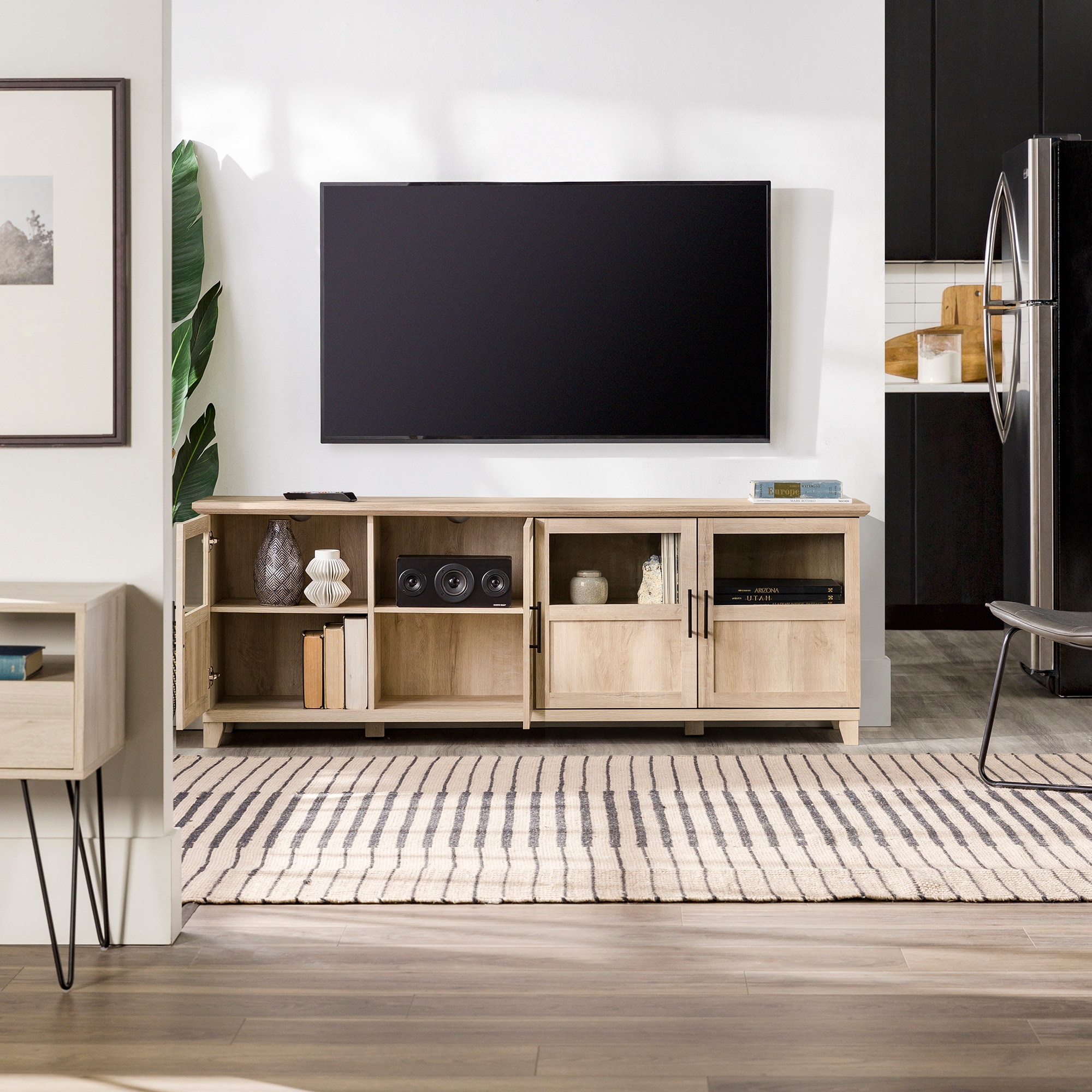This square, indoor photograph, measuring approximately 6 inches by 6 inches, captures a modern, clean-lined living space illuminated by daylight. The image unfolds from left to right across three distinct rooms, unified by continuous light brown wooden plank flooring that shifts orientation in the kitchen area, creating a visually appealing contrast. 

Starting from the left, in the foreground room, a white wall features a framed photograph above a petite wooden table. This flows into the central room, dominated by a light wood TV console with dual sets of cabinets; one side reveals vases, books, and a speaker, while the closed side subtly hints at additional storage. Atop the console, a black remote control rests on the left, and a blue and brown book lies on the right beside a large black flat-screen television mounted on the wall. A visually striking black-and-white rug, reminiscent of piano keys, stretches across the floor in front of the console.

The second room's right wall holds a flat-screen TV above the light wood cabinet, accompanied by a tall green potted plant to its left. To the far right, the kitchen becomes visible with black-painted cabinets, a white tile backsplash, and a gleaming stainless steel refrigerator, surrounded by a sleek, modern aesthetic.